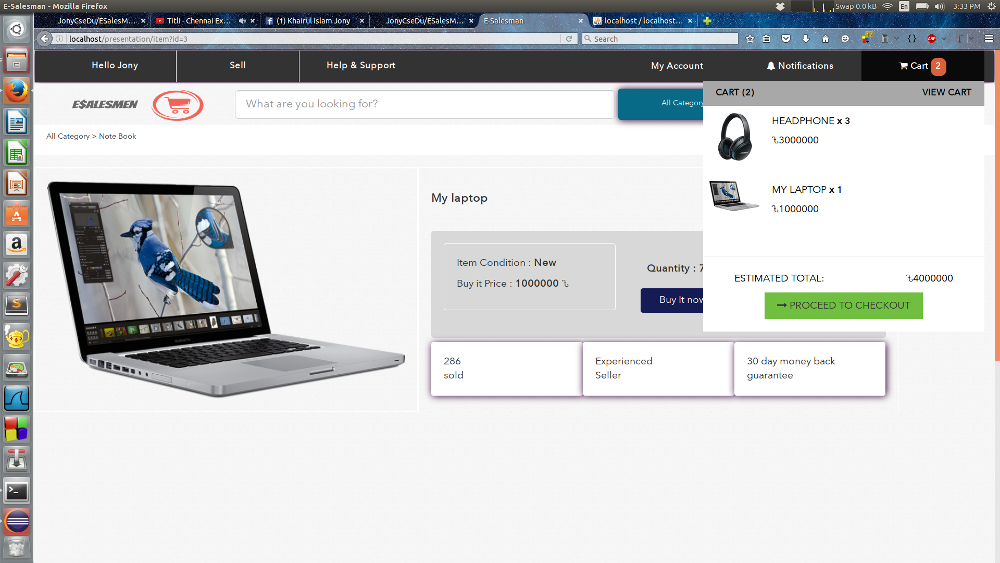The image depicts a webpage from an e-commerce site labeled "e-salesman-mozilla-foxfire," shown on a silver-gray laptop screen. The laptop, which has a sleek design with black keys and a centered trackpad, displays a vibrant image of a Blue Jay. The website is personalized, addressing the user as "Hello Johnny" in the upper left corner.

In the online shopping cart, Johnny has selected three sets of headphones and one laptop, as indicated by "headphones x3" and "my laptop x1". The total cost of the items in the cart amounts to a non-U.S. currency value of 4,000,000, as displayed on the page. A green "Proceed to Checkout" button is prominently featured, inviting Johnny to finalize the purchase.